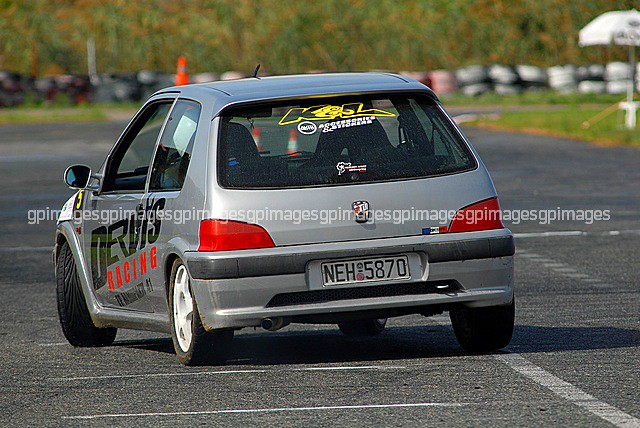The image depicts the back of a gray hatchback racing car, prominently marked with various logos and inscriptions. One distinctive black and red logo on the driver's side door features the word "racing" in red, though the black text remains unreadable. The rear windshield displays a yellow logo with some white information below it that's also not legible. The car, whose white license plate reads NEH5870, is driving across a parking lot with visible parking spaces, accompanied by an orange safety cone positioned ahead. The rims are white, adding a striking contrast to the car's gray body. Surrounding the scene is a slightly blurred green grassy area with what appears to be a hedgerow and possibly a stack of tires. Overlaid across the entire image, including across the car and the background, is a watermark that reads "GP Images" repeatedly.